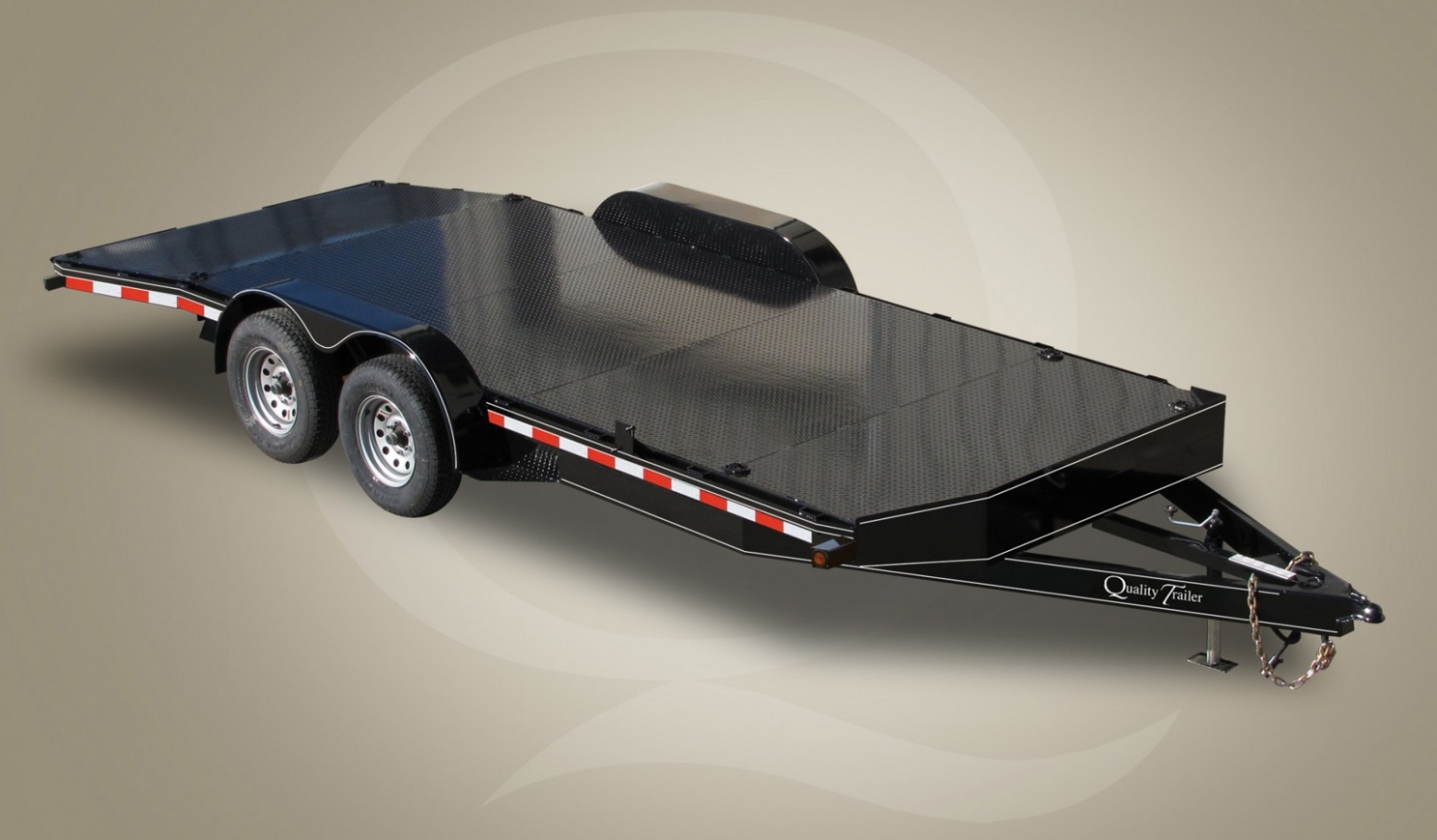This horizontally aligned rectangular image showcases a detailed view of a flatbed trailer against a digitally edited, gradient background transitioning from light gray in the center to a darker shade towards the edges. Central to the backdrop is a faint, stylized letter "Q" formed by a circle and a swirling line. The trailer, designed for attachment to a pickup truck or a car, is depicted from an elevated angle, emphasizing its diagonal placement with the hitching part located in the lower right corner and the rear end stretching towards the upper left.

The flatbed of the trailer is a solid, glossy black with a textured surface, offering both reflectivity and durability. The rear half of the flatbed has a subtle blue tint. Along the right side, there's a prominent stripe consisting of alternating red and white rectangular patterns, designed to be reflective for better visibility. The trailer features two black wheels on the right side, housed in curved black wheel wells, with a matching pair implied on the unseen side.

A sturdy chain wraps around the front V-shaped bars of the hitching post, which bears the text "Quality Trailer" in bold white letters. The prominent use of colors in the image includes black, white, red, and silver, particularly notable in the rim of the tires and the chain. The photograph seems to serve an advertisement purpose, showcasing the trailer's build quality, design details, and potential for various uses, such as transporting equipment, tools, or even a small boat like a canoe.